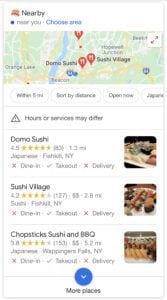This is a very low-quality, blurry screenshot seemingly from a mobile app, likely Google. The background is predominantly white. In the top left corner, in black font, it reads "Nearby." Beneath that, there's a black dot followed by the text "Near you." Next, "Choose area" is written in blue font. Below this, there appears to be a roadmap, most likely from Google Maps, with three red pins marking specific locations.

Directly beneath the map, the text "Sort by distance" can be seen, followed by some other unreadable entries, one of which possibly says "Japanese." Further down, there is a black rectangle with an exclamation point, alongside a message stating "Hours or services may differ."

Below this warning, there is information about a restaurant named "Demo Sushi." It has a rating of 4.5 stars and is located 1.3 miles away. The details state "Japanese, Falkill, New York." The dining options are indicated as Dine-in: No, Takeout: Yes, and Delivery: No. To the right of this information, there's a blurry image of a plate with some food on it.

Below "Demo Sushi," another restaurant is listed: "Sushi Village," which has a rating of 4.2 stars. It is located in Fox Hill, New York. The dining options noted are Sushi: No, Dine-in: Yes, Takeout: No, and Delivery. There is an accompanying image to the right depicting a plate with brown nuggets of food.